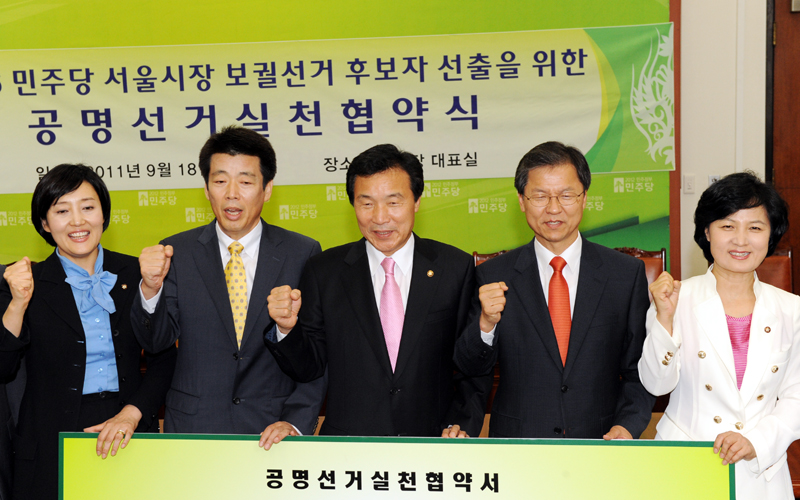A group of five formally dressed Asian individuals stand behind a podium, each with their right fists raised in front of them and their left hands resting on the podium. From left to right, the group includes a woman with short dark hair dressed in a blue blouse and a black jacket; a man in his 40s with short black hair, wearing a blue suit and a yellow tie; a slightly shorter man in his 50s with dark hair, dressed in a dark suit; a bespectacled older man wearing a dark suit and a red tie; and another woman in her 30s with dark short hair, wearing a white jacket over a pink shirt. All hold a large light green sign with Asian lettering at the top, and behind them hangs a similarly colored banner adorned with Asian writing in dark blue.